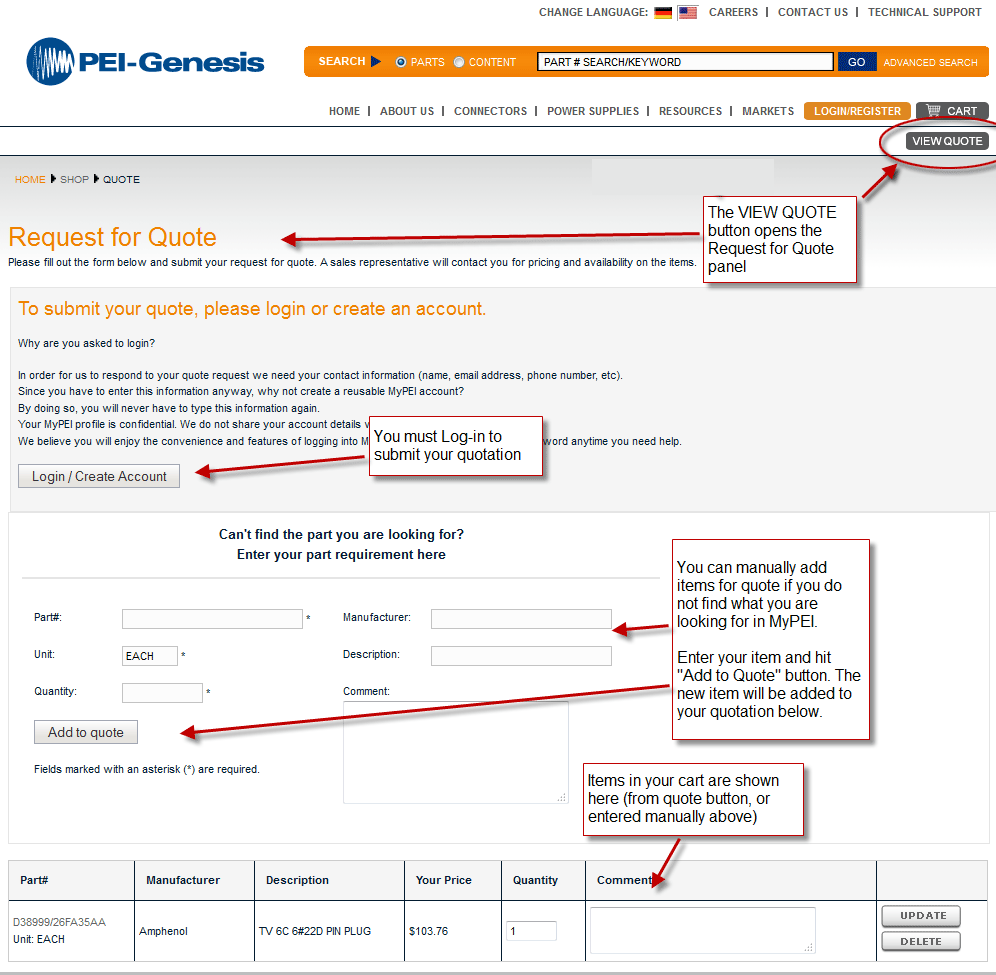The image is a screenshot of the PEI-Genesis website. At the upper left-hand corner, "PEI-Genesis" is displayed prominently. Just to the right of this label, a search bar and search button are located on an orange bar, enabling users to search for products or information.

Directly beneath the orange bar is a right-justified menu bar, featuring various navigation links. Toward the far right of this menu bar, there's a "Login/Register" button. Beside it, circled in red, is a "View Quote" button. 

There's also a white box with a red outline and an arrow pointing to the "View Quote" button. Within this box, text explains that the "View Quote" button opens the request for quote panel. Following this, another red arrow points to the "Request for Quote" section, indicating the purpose and functionality of the button.

Additionally, a help instruction overlay is visible, guiding users through the process of using the request for quote feature. The overlay includes another arrow pointing to the "Add to Quote" button, further assisting users in navigating the website.

The overall layout and highlighted instructions convey a step-by-step guide to help users efficiently request a quote on the PEI-Genesis website.